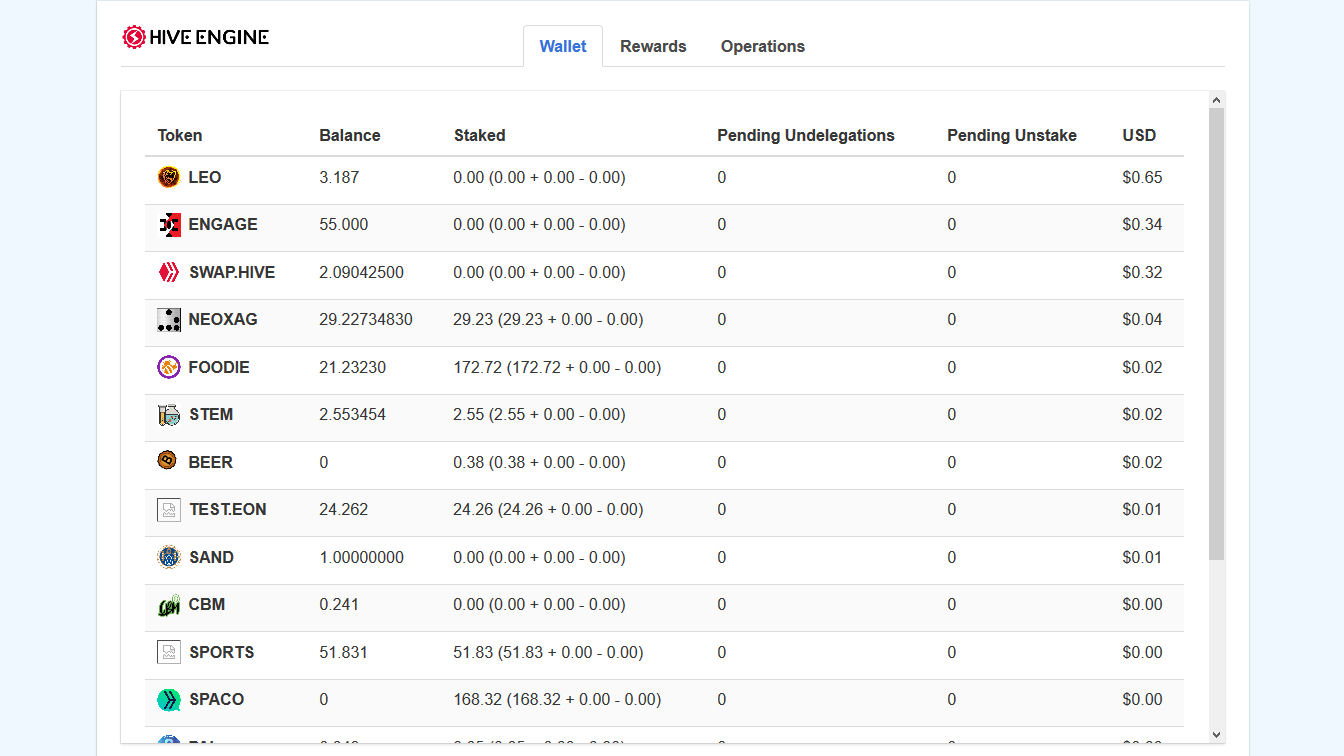The image displays a webpage with a predominantly white background framed by light bluish borders on the left and right. At the top left corner, there is a distinctive red circle with lines radiating from it, encasing an unspecified symbol or sign, alongside the text "Hive Engine" in black. 

Central to the page, the word "Wallet" is highlighted in blue, while "Rewards" and "Operations" appear in black text. 

Below this section, a table is organized into multiple columns marked by headers: "Token," "Balance," "Staked," "Pending on Delegations," "Pending on Stake," and "USD." 

- The "Token" column lists various token names such as Leo Engage and Swap.Hive.
- The "Balance" column contains a variety of numerical values.
- Under "Staked," another set of numerical figures is presented.
- The columns for "Pending on Delegations" and "Pending on Stake" uniformly show zeros.
- The "USD" column displays specific monetary amounts, such as $0.65 and $0.34.